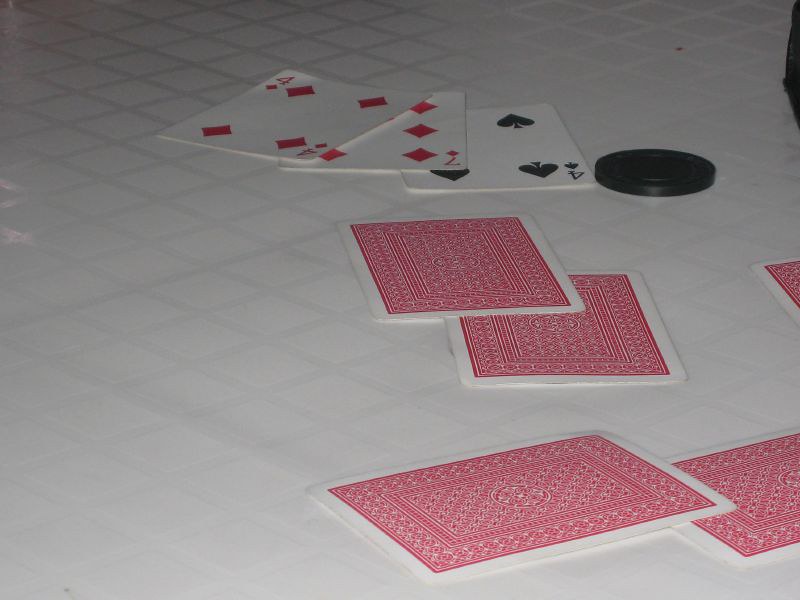An indoor photograph taken in low light conditions depicts a table, likely with a white patio surface or perhaps covered with a white tablecloth adorned with a subtle pattern of faint gray lines forming square shapes. The primary focus lies slightly right of center and towards the background, where seven playing cards are arranged. Three cards positioned sequentially from top to bottom display the four of diamonds, seven of diamonds, and four of clubs. Adjacent to the four of clubs on the right, a solitary black poker chip is visible.

In the center-right of the image, two cards lay face down, showcasing a deck's intricate red back pattern. In the foreground, a single face-down card is diagonally positioned with its top edge pointing towards the right and its bottom edge towards the lower left, slightly overlapping another card lying in a similar orientation but partially cut off by the photograph's right edge. Additionally, at the upper center-right edge, the corner of another card peeks into view, accompanied by a hint of a black object in the image's extreme upper right corner. The photograph is well-focused but exhibits a slightly dark ambiance due to the low light.